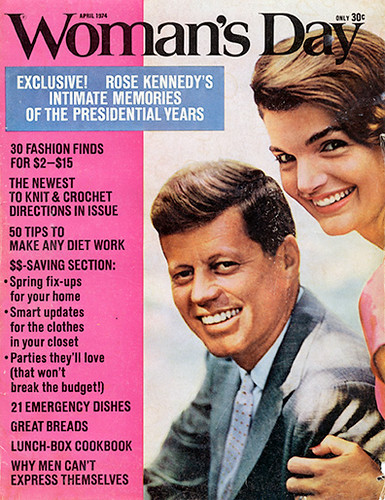This detailed caption synthesizes the contributions from all three descriptions provided:

"Cover of the April 1974 issue of Woman's Day magazine, priced at 30 cents. The prominent black Woman's Day logo spans the top of the cover, with 'Only 30 cents' noted above the 'Y'. To the left, a blue box with white text announces, 'Exclusive! Rose Kennedy's intimate memories of the presidential years'. Taking up the right side is a smiling photograph of President John F. Kennedy and Jacqueline Onassis; she is wearing a pink blouse and has her left hand placed on his left shoulder, while he is in a gray suit with a blue tie.

A pink column runs down the left side of the cover, listing the magazine's features in blue text: '30 fashion finds for $2 to $15', 'The newest in knit and crochet directions', '50 tips to make any diet work', 'Dollar-saving section', 'Spring fix-ups for your home', 'Smart updates for the clothes in your closet', 'Parties they'll love that won't break your budget', '21 emergency dishes', 'Great breads', 'Lunchbox cookbook', and 'Why men can't express themselves'. This vibrant cover captures the essence of the era with its informative and varied content."